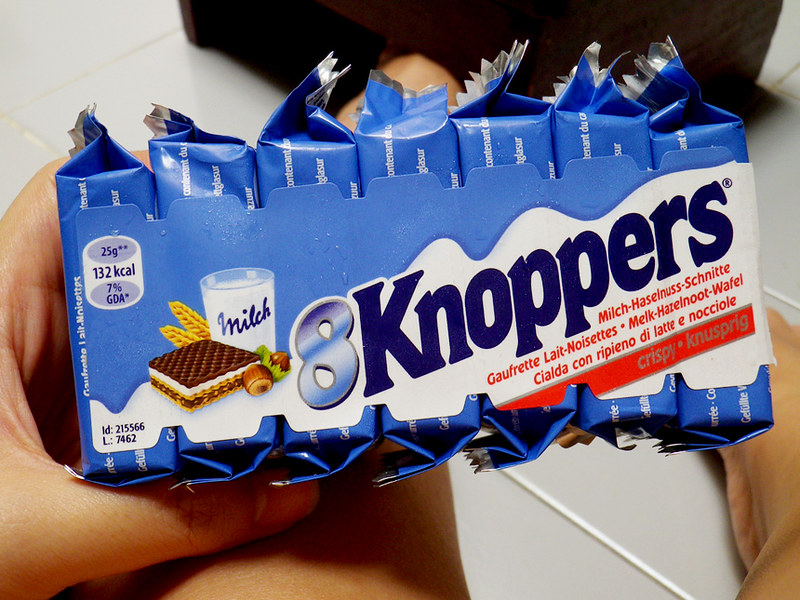The image depicts a packaged snack product called "Knoppers," prominently displayed with the text "8 Knoppers" on the packaging. The package is held by a hand, with a visible fingernail at the bottom and what appears to be part of a leg beneath the hand. The background consists of a white tiled surface and possibly a kitchen counter. The packaging itself is a seven-pack of individually wrapped snacks in a blue wrapper with silver edges. 

To the left of the text "8 Knoppers," there's an illustration of the snack: a multi-layered wafer with a chocolate layer, a white creamy layer, and another cookie layer interspersed with chocolate and hazelnut pieces. The illustration also includes a glass of milk, some wheat stalks, and a hazelnut. The text on the package includes several non-English words, possibly German, such as "Milch," "Haselnuss," "Schnitt," "Garfrucht," and others. The package also notes the snack's nutritional information, indicating 132 calories and 7% GDA.

The setting is a domestic environment, implied by the white tile and possibly a wooden table seen in the background. The snack is designed to appeal with its blend of creamy and crunchy textures, visualized through the detailed illustration on the package.